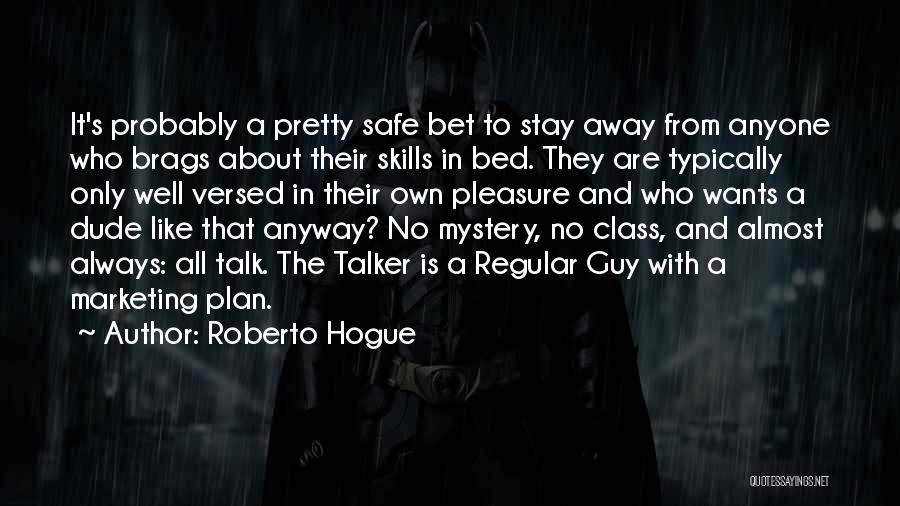The image is a predominantly dark and blurry cityscape scene with a rainy ambiance. The focal point of the scene features a man dressed as Batman, discernible mainly by his signature bat belt, although his upper body and face are obscured by text. Above the figure, in white font, is a prominent quote that reads: "It's probably a pretty safe bet to stay away from anyone who brags about their skills in bed. They are typically only well-versed in their own pleasure, and who wants a dude like that anyway? No mystery, no class, and almost always all talk. The talker is a regular guy with a marketing plan." The quote is attributed to Roberto Hogue, and the bottom right corner of the image bears the watermark "quote essayings.net". The backdrop of this text consists of various shades of black and gray, contributing to an abstract yet vaguely Batman-themed image. The text occupies roughly three-quarters of the image, making it the central focus.